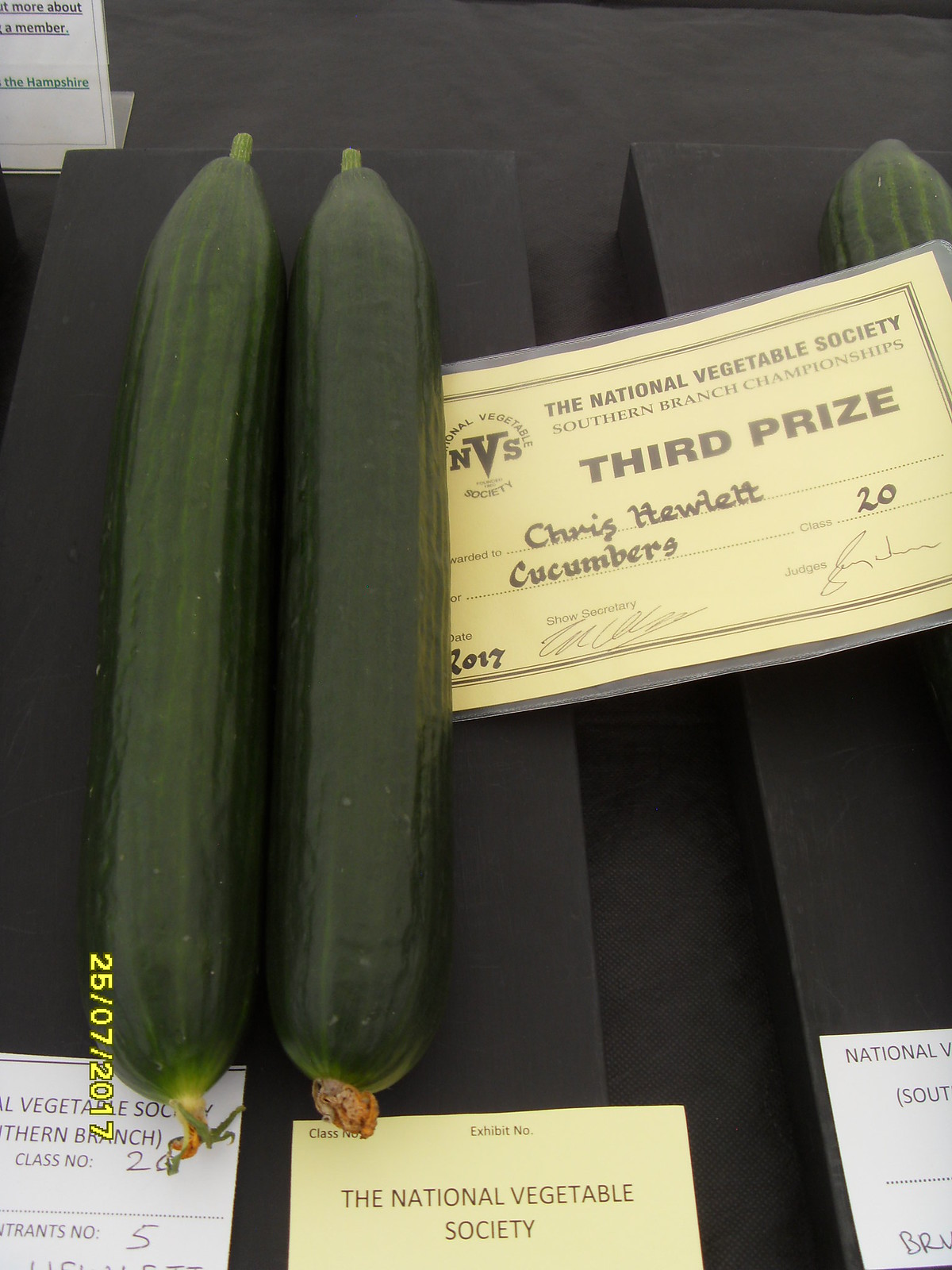The image captures a scene from a cucumber judging competition, featuring three cucumbers displayed on a black table. Two cucumbers are positioned vertically on the left, with a third cucumber placed to the right. A laminated card, partly visible, lies below them, bearing the text: "National Vegetable Society Southern Branch Championships, Third Prize, Chris Hewitt, Cucumbers, Class 20," along with the date, July 25, 2017. Additional cards with cut-off text are beneath this main card. The color palette of the image comprises the green of the cucumbers, the yellow and white of the cards, and the black of the table and text.